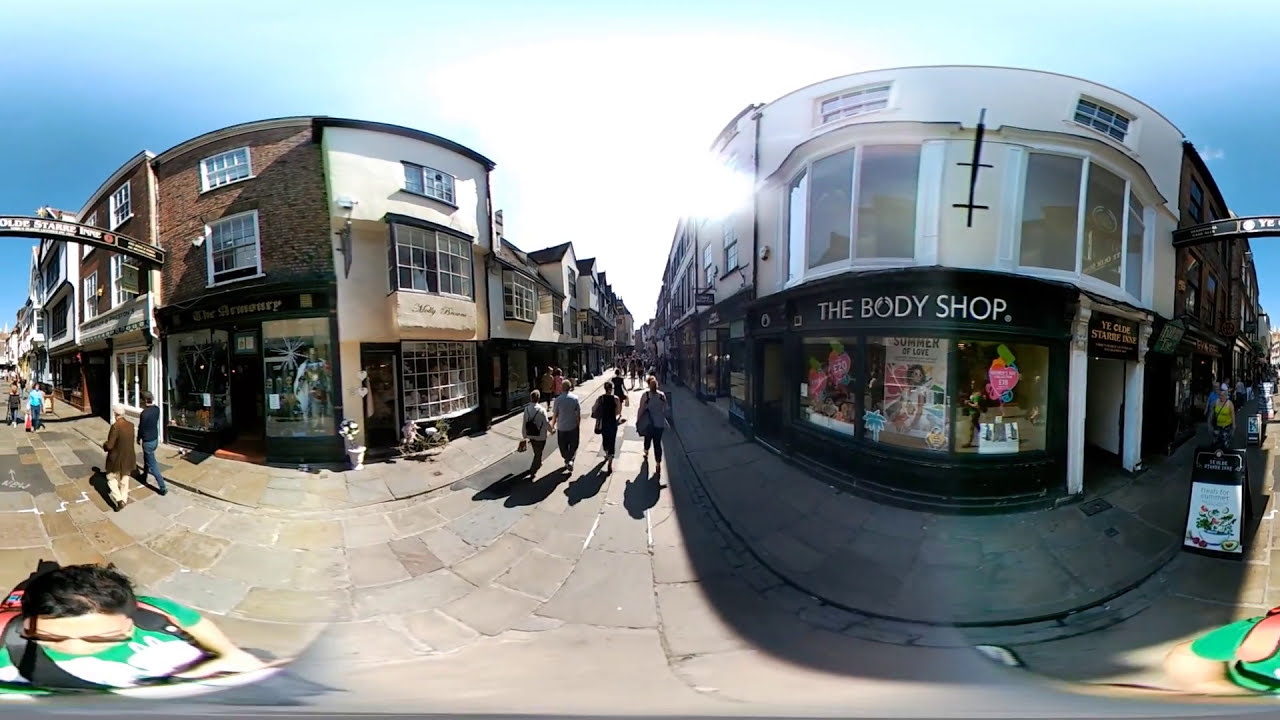This image captures a wide panoramic view of a bustling urban shopping district, possibly taken with a 360-degree or 180-degree camera, as indicated by the warping along the bottom edges. The main focus is a cobblestone street that stretches away from the viewer toward the horizon. This central thoroughfare, along with two intersecting streets branching off to the right and left, is filled with numerous pedestrians, adding vibrant life to the scene.

Flanking the main street are multi-story buildings housing various stores and residences. On the right corner stands a notable establishment with a black and white facade, identified as "The Body Shop," its dark blue exterior adorned with several advertisements. Adjacent to it, a black and white street sign is partially visible.

Further along the streets, although some signage is too distant to discern, a variety of shops with colorful signs suggest a lively commercial area. Indie fashion boutiques and other small stores line these pedestrian paths, contributing to the area's eclectic charm.

In the foreground, the viewer’s perspective is anchored by distorted images of people—one woman in a green shirt and sunglasses on the bottom left and another figure on the bottom right. The sky frames the scene with hues of blue in the corners and a bright white glow in the center, likely from the sun's intense brightness.

This detailed composition captures the essence of an active urban intersection, emphasizing its vibrant commercial activity and the close-knit architectural style of the neighborhood.